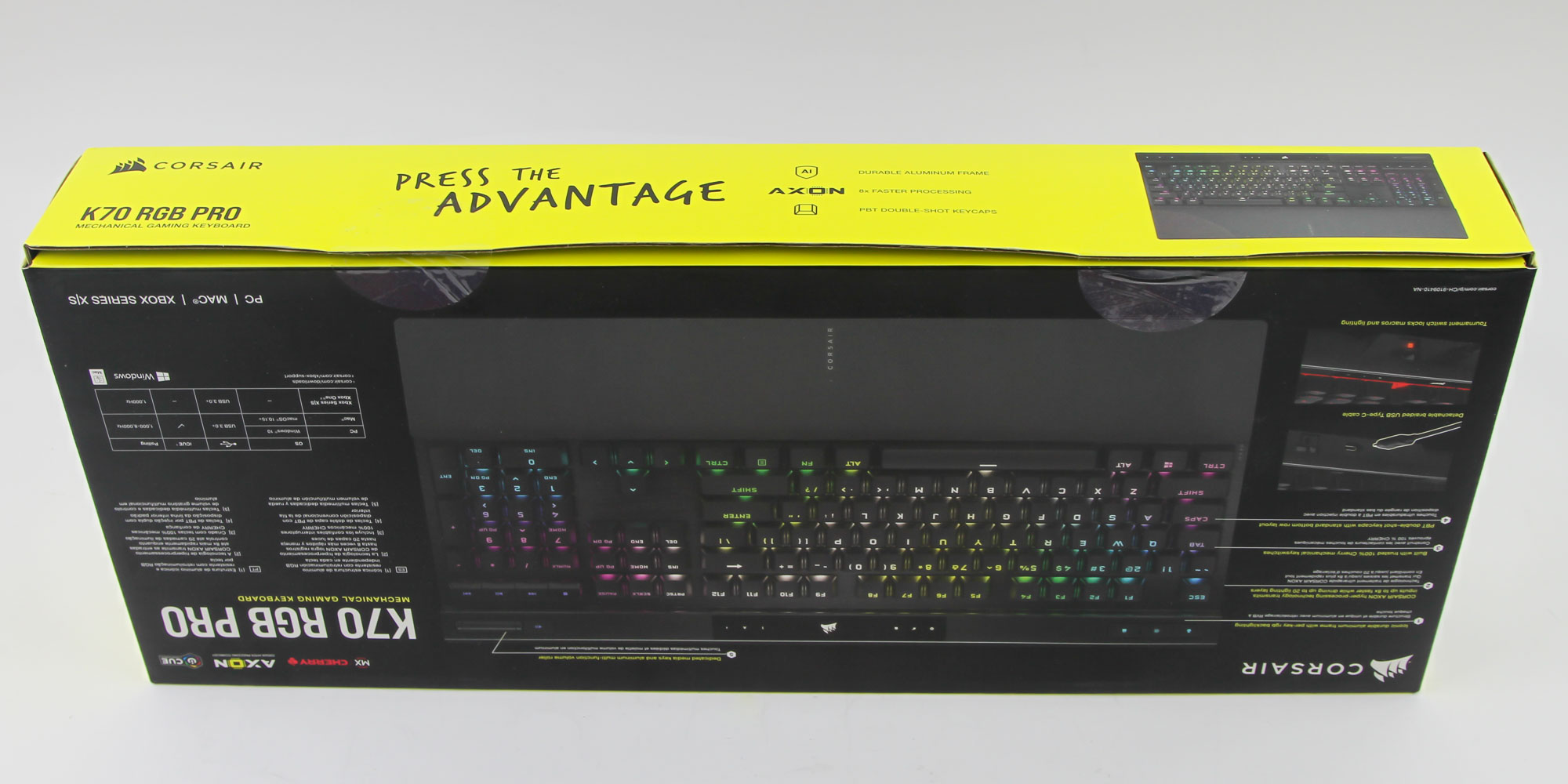The image showcases a boxed keyboard, primarily featuring a vibrant yellow top and black sides. Prominently displayed in the center of the box is the phrase "Press the Advantage," accompanied by the brand name "AXON." At the bottom left corner, the model is specified as "K70 RGB Pro." The keyboard itself is black, with keys that illuminate in a spectrum of rainbow colors, suggesting customizable RGB lighting.